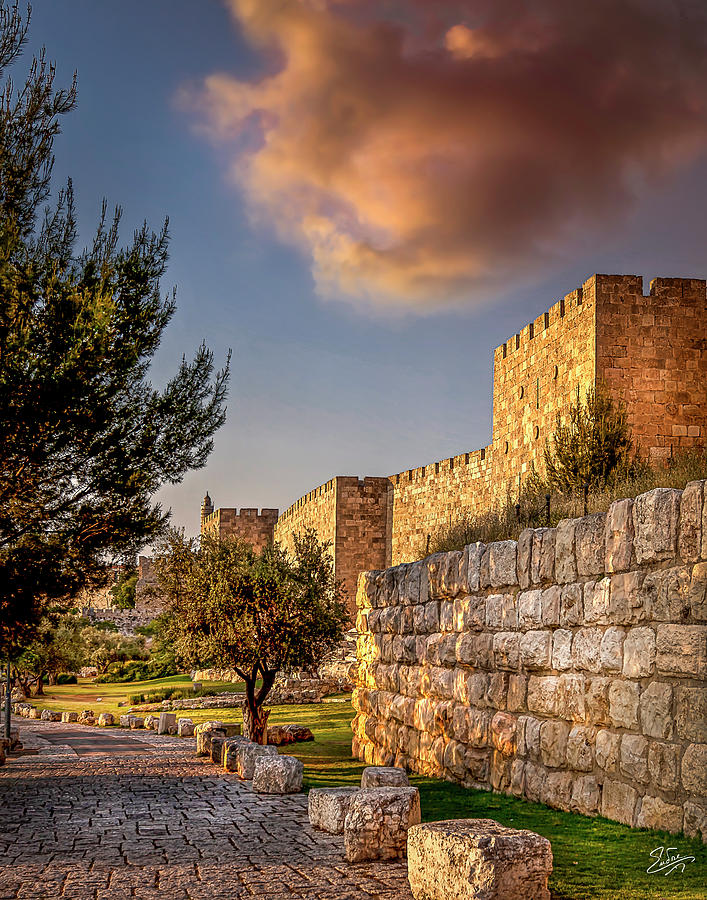The image captures an outdoor scene set in a historic city, prominently featuring a medieval castle or fortress. The right side of the image reveals the back side of this structure, characterized by tall, well-aligned stone walls in varying shades of tan with highlights of white. Notably, the upper section of the wall exhibits a dental molding pattern with outlooks at regular intervals. The wall, which initially appears to hold back a hill or mountain, extends up to two stories high.

The foreground showcases a stone ledge adorned with greenery and small trees. Below this ledge, a meticulously paved stone walkway leads through the scene. This walkway transitions to a cobblestone roadway, lined with large stones, flanked by a tall, full tree on the left and a shorter, equally lush tree on the right. The circle around the tree on the left appears to be a paved sitting area, harmonizing with the larger stones.

The sky, a clear blue with a touch of golden hue on one visible cloud, suggests the time is either sunrise or sunset, casting a tranquil light over the scene. This careful alignment of natural elements against the backdrop of historic architecture creates a unique and vivid image of a beautifully preserved area, possibly an entrance or courtyard within the castle or fortress walls.